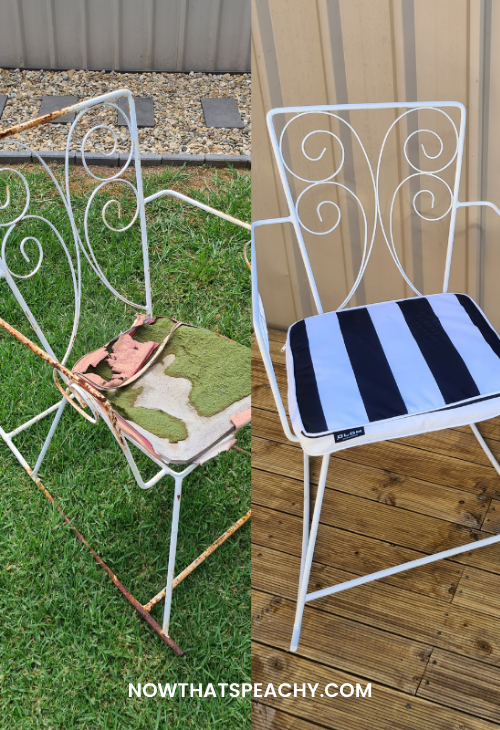The image is a vertically split before-and-after photograph, showcasing the dramatic restoration of a metal chair. On the left side, the chair is depicted in a severely dilapidated state, with extensive rust covering its once white iron frame and a disintegrated, cushion-less seat. The chair rests on a grassy area with a gravel path and some stones in the background, possibly near a shed or garden fence. This neglected piece appears beyond repair, with peeling paint and rust ranging from light to dark brown.

In stark contrast, the right side reveals the same chair after a meticulous restoration. The metal frame has been rejuvenated with a pristine white finish, entirely free of rust. The seat now boasts a fresh, upholstered cushion featuring dark blue and light blue stripes. The transformed chair is positioned indoors on a hardwood floor, against a backdrop with gray, beige, and dark brown striped wallpaper. At the bottom of the image, the text "NowThat'sPeachy.com" suggests that this impressive transformation was carried out by a professional furniture refreshing service.